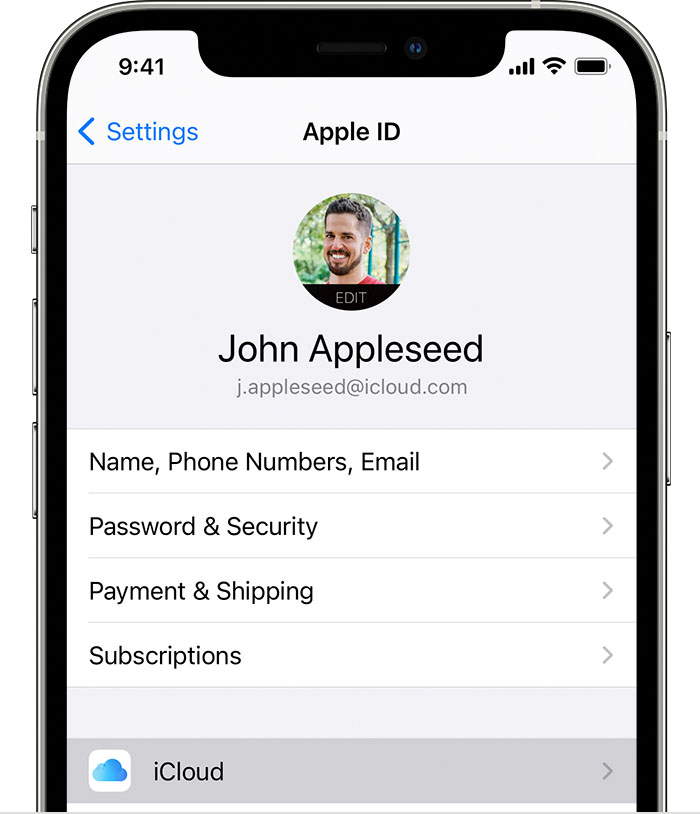A close-up photo of a silver iPhone screen displaying the Apple ID settings page at 9:41 AM. The status bar at the top shows full WiFi signal, a fully charged battery, and the time in blue text. The phone's settings screen features various options in a list below a profile picture of a smiling individual with a tray in the background. The Apple ID displayed is "JohnAppleCJ.AppleCJ@icloud.com." The list of options includes "Name, Phone Numbers, Email," "Password & Security," "Payment & Shipping," "Subscriptions," and "iCloud." There is also a gray and blue cloud icon representing iCloud. Alongside the screen, the phone's physical buttons, such as the volume up and volume down controls, are visible on the edge of the device.